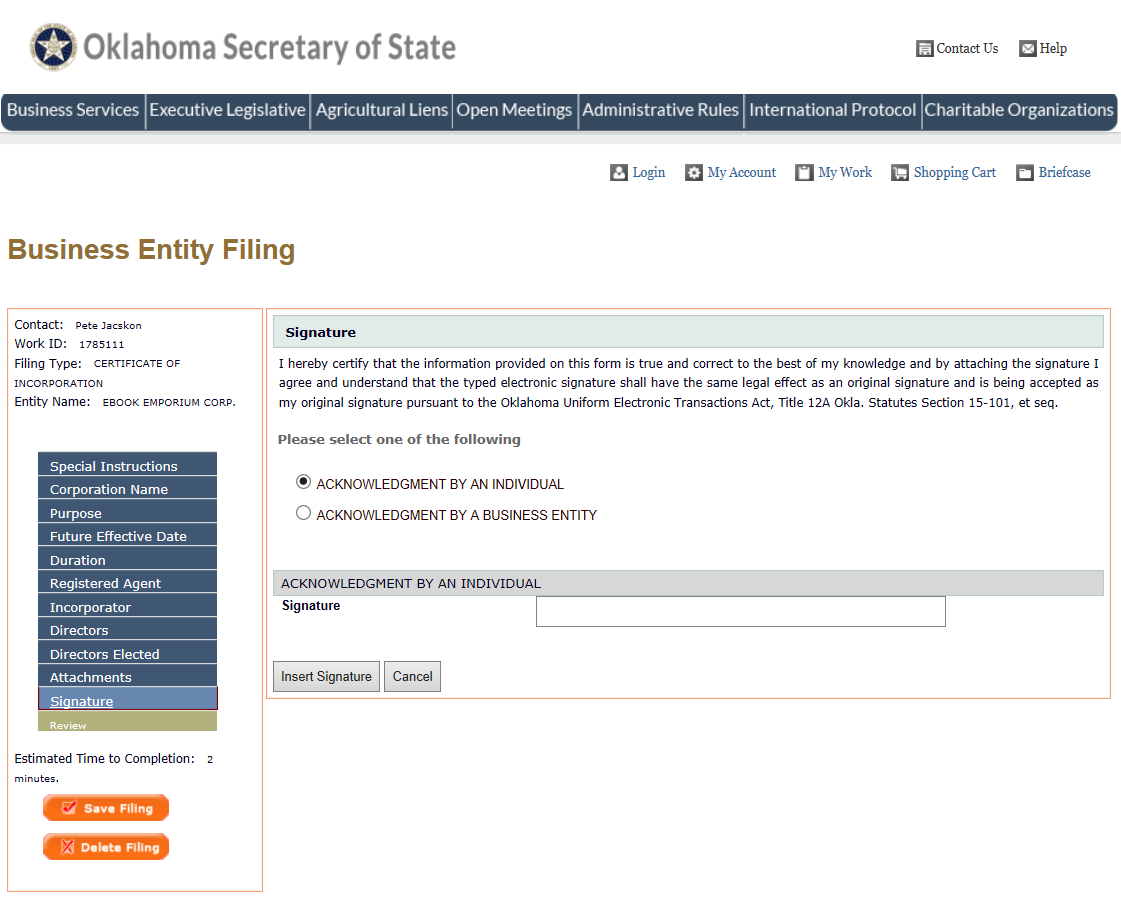The image is a screenshot from the Oklahoma Secretary of State’s website, specifically displaying various service options and a digital signature section. In the upper portion of the image, there are navigational tabs labeled "Business Services," "Executive," "Legislative," "Agricultural Liens," "Open Meetings," "Administrative Rules," "International Protocol," and "Charitable Organizations." The lower portion contains a digital signature form. The form includes a notice stating: "I hereby certify that the information provided on this form is true and correct to the best of my knowledge, and by attaching the signature, I agree and understand that the typed electronic signature shall have the same legal effect as an original signature and is being accepted as my original signature pursuant to the Oklahoma Uniform Electronic Transaction Act, Title 12A, Oklahoma Statute, Section 15-101 et seq." There is a selection marked "Acknowledgement by an individual," while "Acknowledgement by a business entity" is unselected. The interface features an "Insert Signature" button and a "Cancel" button.